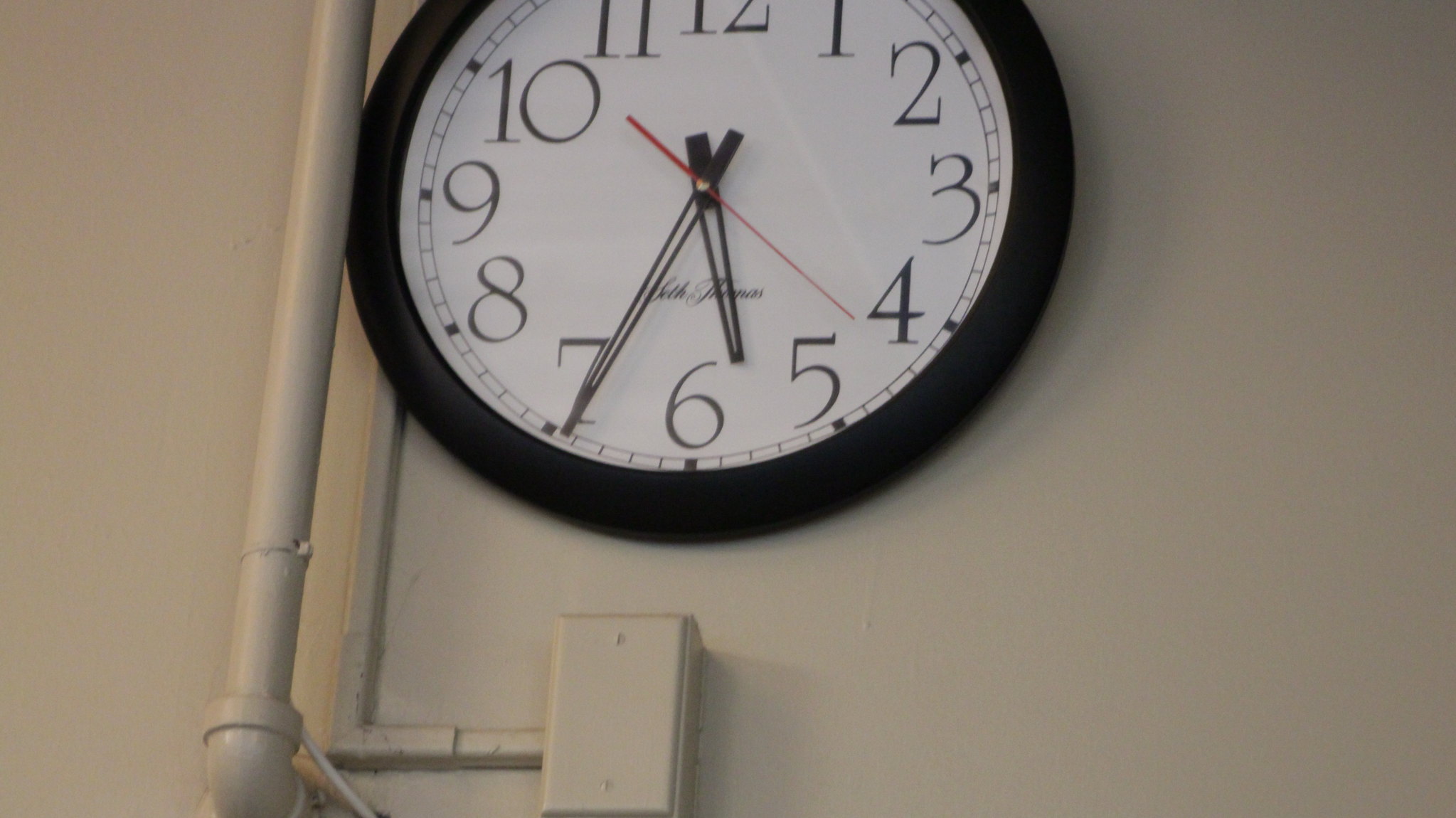This is a color photograph taken indoors, featuring an older, slightly grainy quality. The image is rectangular and wide, focused on a portion of a smooth, off-white painted wall. Centrally positioned, though slightly towards the upper middle, is a round black wall clock. The clock has a white clock face with black numbers and black hour and minute hands; a thin red second hand also ticks around the white face. Surrounding the clock are fine black dash marks in a circular pattern. The bottom portion of the clock shows some indistinct writing, possibly a brand name. 

To the left of the clock, a white industrial-looking pipe extends vertically, with another white electrical cord resting atop it. Underneath the clock, a white, industrial-looking box, mounted to the wall, is visible. Soft circular shadowing from the clock can be seen cast against the wall, adding to the depth and texture of the composition. The overall neutral tones and practical elements give the scene a utilitarian aesthetic.